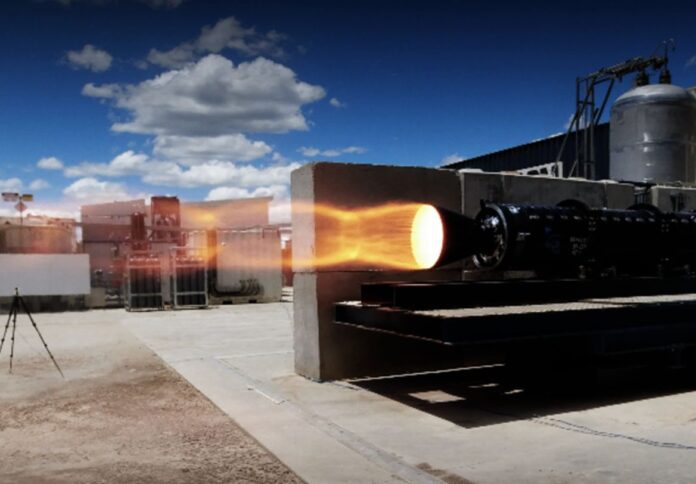This daytime outdoor color photograph showcases a rocket testing facility under a rich blue sky adorned with fluffy white clouds. Dominating the right side of the image is a low dark gray concrete wall, in front of which sits a flatbed tractor bearing a black cylindrical missile pointed towards the right. From the missile's exhaust ring, a brilliant circle of white light followed by yellowish-orange elliptical flames radiates powerfully to the left side of the image. Adjacent to the missile, a vertical cylindrical silver tank stands on a concrete platform, topped by a metal arm, suggestive of industrial apparatus. The background juxtaposes a hard-packed brown dirt ground with a gray concrete flooring, all enclosed by substantial grey concrete blocks, highlighting the industrial setting. Scattered structures and a tripod with a white board further enrich the scene, creating a vivid and detailed portrayal of the facility.